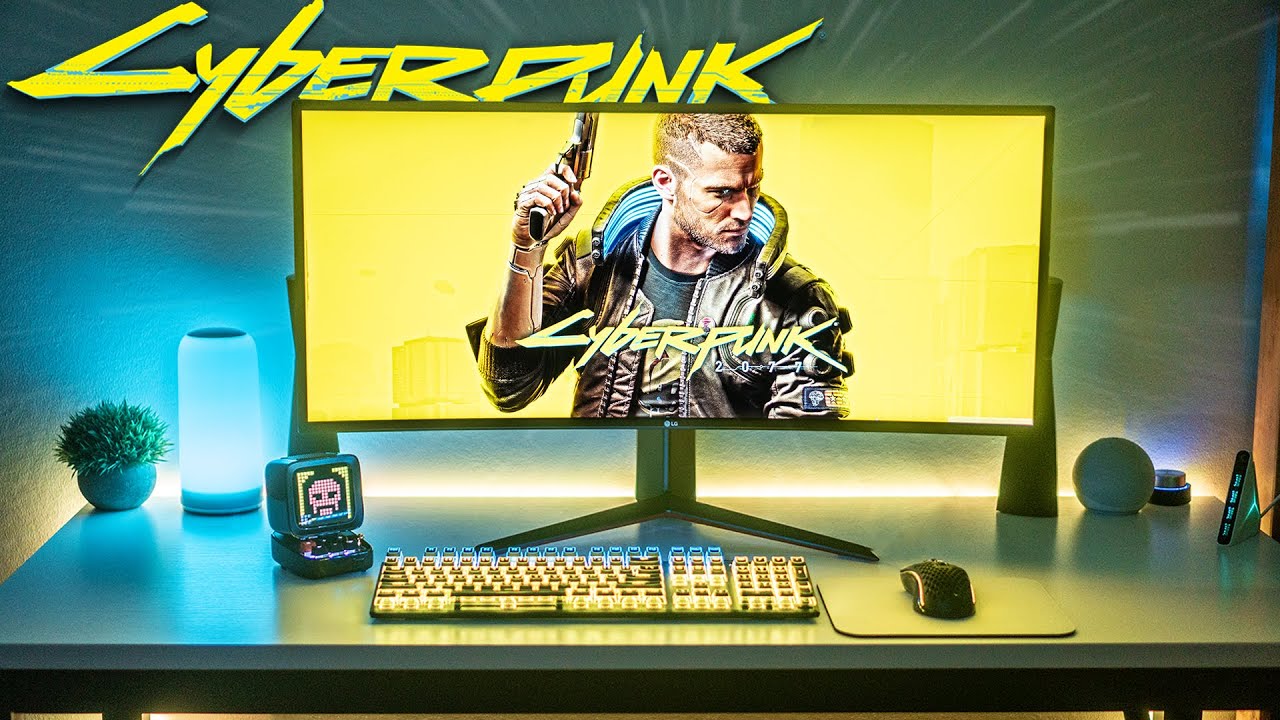The full-color image, a blend of photograph and digital enhancement, is horizontally rectangular without any specific border or background. At the bottom of the image, a clean and neat white desk is visible, giving the impression of sitting at that table. Central to the image, a large computer monitor displays a young, white man with short hair, dressed in a brown leather jacket and holding a gun. The screen features a yellow background with the title "Cyberpunk 2077" prominently displayed across the man's chest. Above, on the wall behind the monitor, the word "Cyberpunk" appears again in the same yellow lettering. In front of the screen, on the desk, there is a keyboard and mouse neatly placed. To the right of the monitor, various knick-knacks are visible, adding a personal touch to the space. In the upper right corner, a small green plant next to a glowing blue light provides a subtle contrast, while in the left corner, another plant and a round object are present, contributing to the overall organized and simplistic aesthetic of the scene.